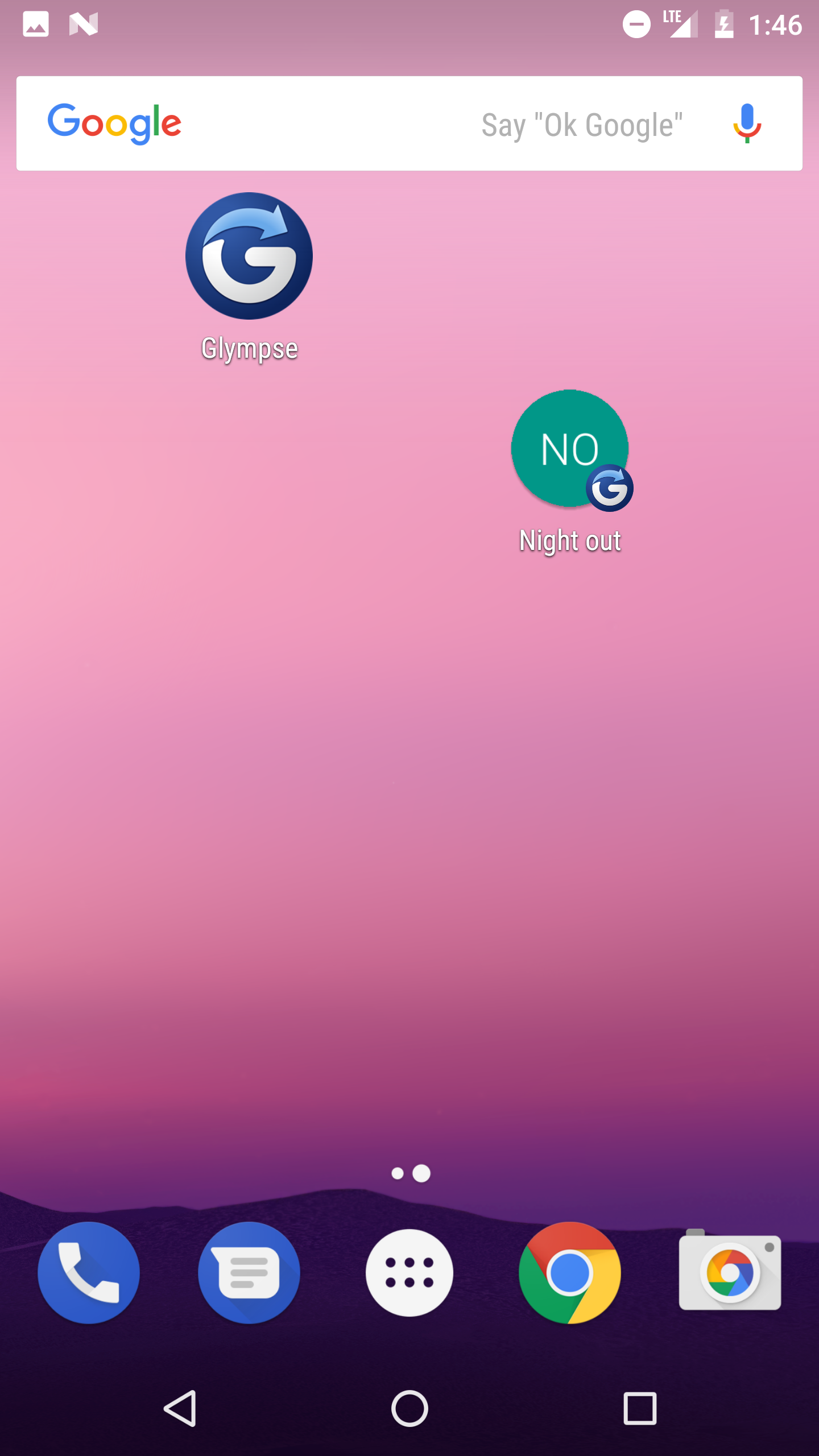This screenshot captures the home screen of an Android device, recognizable by its distinct navigation bar at the bottom featuring a left-facing arrow button, a circular home button, and a square apps button. The device is currently on the second page of the home screen, indicated by the two dots at the bottom where the right dot is highlighted. This suggests that swiping left would reveal the main home screen.

The wallpaper is a minimalistic depiction of a mountain peak at sunset. The mountain silhouette lies at the bottom of the screen, where the main icon bar resides, and the sky above is adorned with gradient hues of purple and pink.

At the top of the screen, a Google search bar is prominently displayed, complete with a microphone icon for voice search through the "OK Google" function. Below this search bar, two app icons are neatly positioned. The first app, named Glimpse, has a blue icon with a stylized "G" inside it. Adjacent to it, the second app is titled Night Out, represented by a green icon with the initials "N-O." Interestingly, the Night Out icon features a small Glimpse icon at its bottom right corner, indicating some form of integration or connection between the two applications.